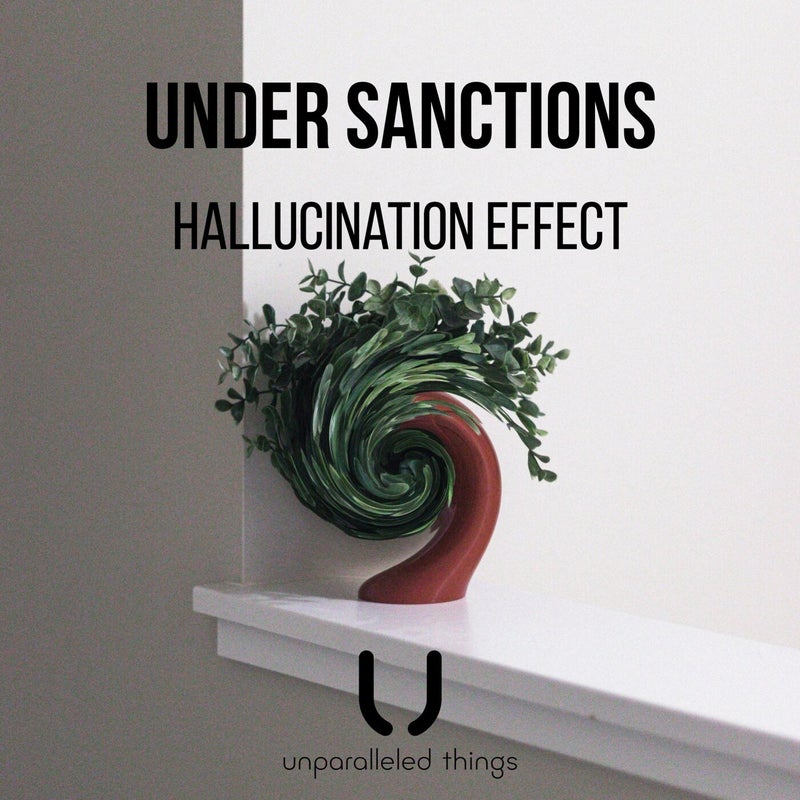The image is a color photo that appears as a poster, featuring a white shelf mounted on a wall with varying shades of gray and beige. Positioned on the shelf is an ornate, curvy vase with a bright red base and green leaves sprouting and twisting around it, creating a dynamic, spinning effect that adds to the surreal theme of the poster. At the top of the image, bold black text reads "Under Sanctions," with "Hallucination Effect" written just below in smaller black letters. At the bottom, a distinctive logo composed of two vertically curved lines is accompanied by the text "Unparalleled Things," also in small black letters.